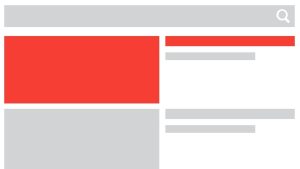The image displays a minimalist website layout characterized by its clean lines and muted color scheme. At the very top, a solid gray banner stretches across the width of the screen, devoid of any text or imagery except for a small white magnifying glass icon situated at the far right, suggesting a search function. 

Below the banner, the content area is divided into two columns. The left column features two vertically-aligned squares: the top square is red, and directly beneath it is a gray square. 

To the right of these squares, in what appears to be the right column, lies a long red rectangular box. Positioned below this box is a gray rectangular box, about three-quarters the length of the red one above it. 

For the right-hand section of the content area, aligning with the left column's gray square, there is another long gray rectangular box. Directly below this is a secondary gray rectangular box, approximately two-thirds the length of the one above it. 

The overall layout is simplistic with no additional text or graphical content, highlighting the structural elements of the website design.